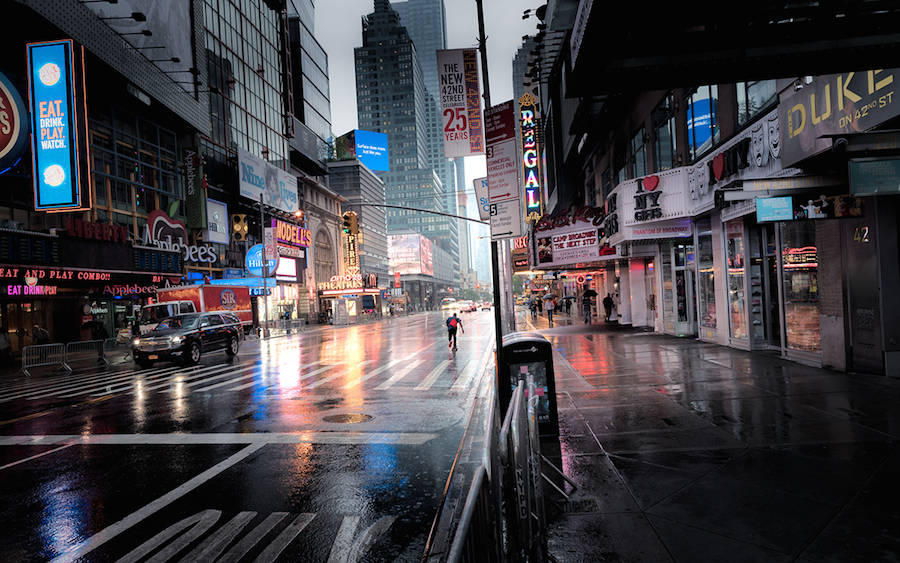This image captures a bustling city street in downtown New York City during the evening. The road, which runs centrally through the image and diagonally towards the bottom left, appears wet and reflective, suggesting a recent rainfall on this overcast day. The photo is taken from the edge of a sidewalk, looking down the length of the street adorned with numerous illuminated businesses and signs.

Prominent establishments include a brightly lit Dave & Buster's with its "Eat, Drink, Play, Watch" sign, an Applebee's, and a Regal Cinema with its vertical, white illuminated sign visible from afar. Other notable businesses are Isle of New York Gifts, Duke on 42nd Street, and a sign announcing "The New 42nd Street, 25 years." There are a few cars parked along the sidewalk, with a black Chevy SUV being the most prominent near the camera. A single vehicle with its headlights on is driving down the street, which is relatively light on traffic.

Pedestrian activity is present but sparse, with a few people scattered along the sidewalks and a man running down the middle of the street, heading away from the viewpoint. Additionally, a skateboarder with a red backpack can be seen using a bike lane. Skyscrapers loom in the distance, completing the dynamic urban backdrop of this iconic New York street.